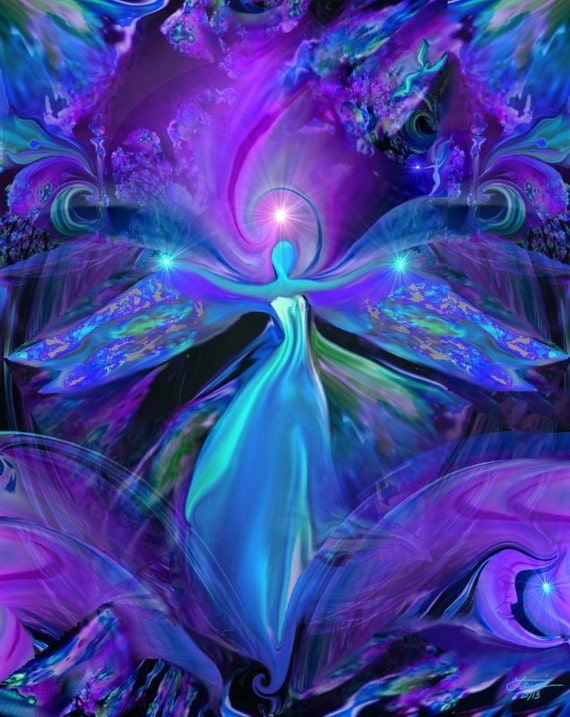This vertically aligned, computer-generated image is a highly artistic and abstract representation, predominantly featuring hues of blue, purple, and touches of green. Central to the composition is the ethereal outline of a figure that can be interpreted as an angel, princess, or fairy. The figure is distinguished by an oval shape for the head, devoid of facial features, and is clad in a flowing white gown that extends from the chest and shoulders. At the tips of her outstretched arms are illuminated white stars. Behind her, vivid purple wings adorned with psychedelic swirls of orange, green, and yellow add to the surreal atmosphere. Hovering above her head is a swirled halo with a central star. The background enhances the mystical quality of the scene with intricate patches of blue and green in the upper corners, complemented by expansive swirls starting from the bottom center, which transition from blue to purple with streaks of darker purple. The overall fusion of colors and elements epitomizes creativity and an abstract sense of wonder.